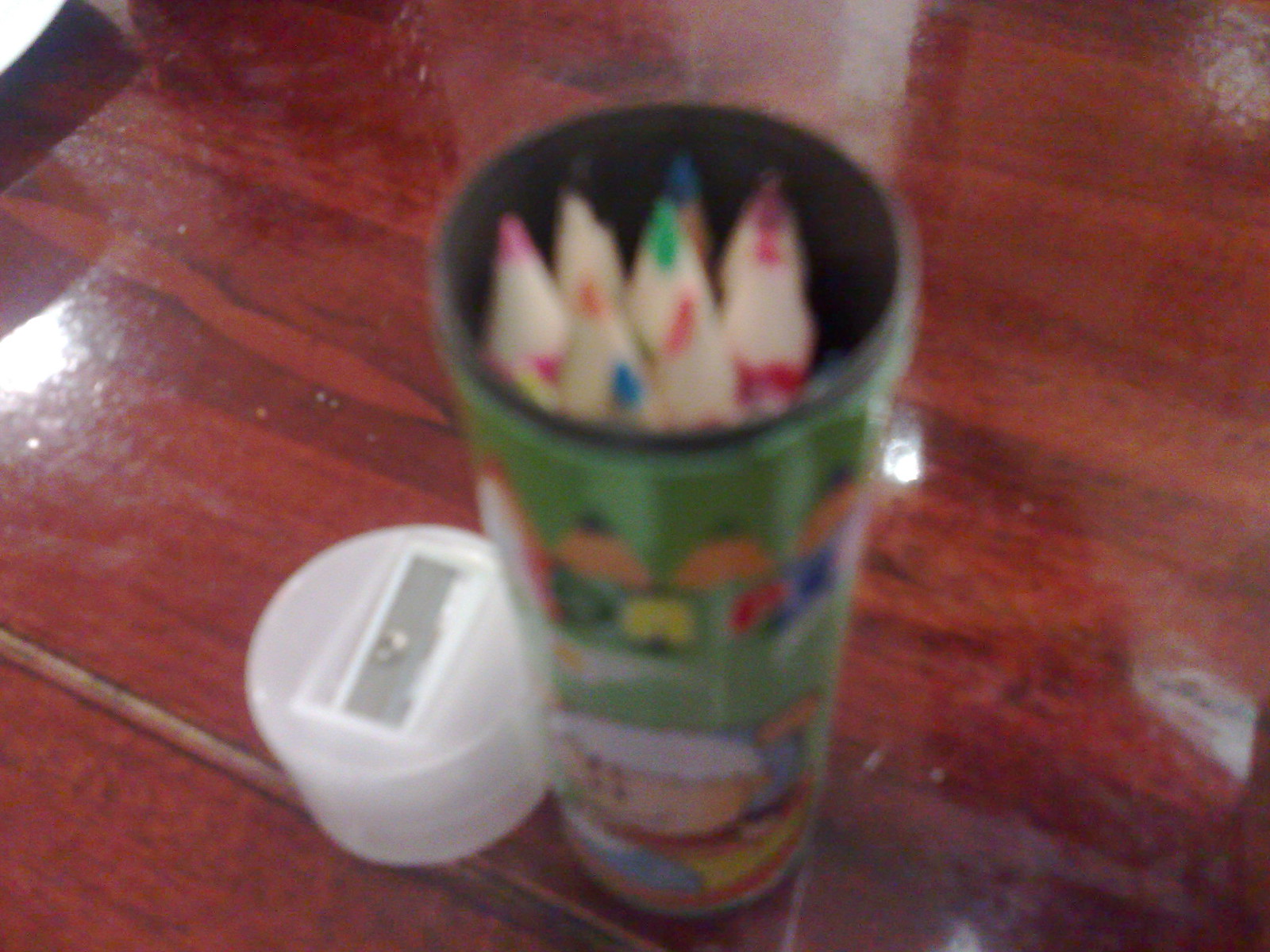On a highly reflective and richly varnished table, likely made of redwood or stained red, sits a green cylindrical container adorned with a cartoonish character featuring white hair. This container, which is either metal or plastic, holds several colored pencils. The pencils include shades of pink, black, blue, red, green, orange, navy blue, and an additional dark red. The green container appears decorated with whimsical drawings, suggestive of pencil tips and possibly additional character features. Beside this container, there is a small cylindrical pencil sharpener that is either white or clear plastic with a silver part on top. The shiny surface of the table reflects various items beyond the frame, adding depth to the blurred and out-of-focus overall image. The emphasis on the table's gleam contrasts with the indistinct details of the colorful pencils and containers, suggesting a picture possibly taken at an isometric 45-degree angle.